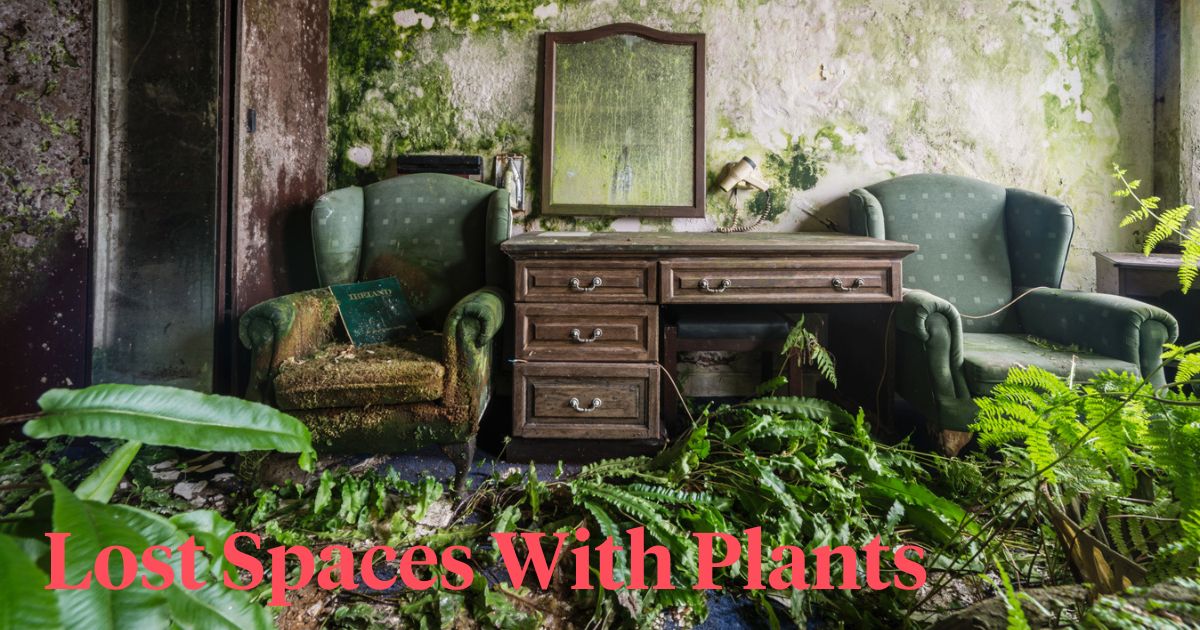In this haunting image, nature has reclaimed an abandoned home, untouched for decades with an open door allowing the wilderness to seep in. The room is consumed by rampant vegetation; vines snake across the floor and climb the walls, which are heavily peeled and encrusted with moss. An old wooden desk dominates the center, flanked by two neglected armchairs, their green polka-dotted upholstery tattered and overtaken by grime and moss. A forlorn mirror hangs on the wall, its surface obscured entirely by moss, reflecting nothing but decay. To the left, an open doorway leads to more unseen ruin, while every surface is a testament to the relentless encroachment of plants. At the bottom of the image, a stark red caption reads, "Lost Spaces with Plants," encapsulating the eerie fusion of abandonment and natural reclamation.